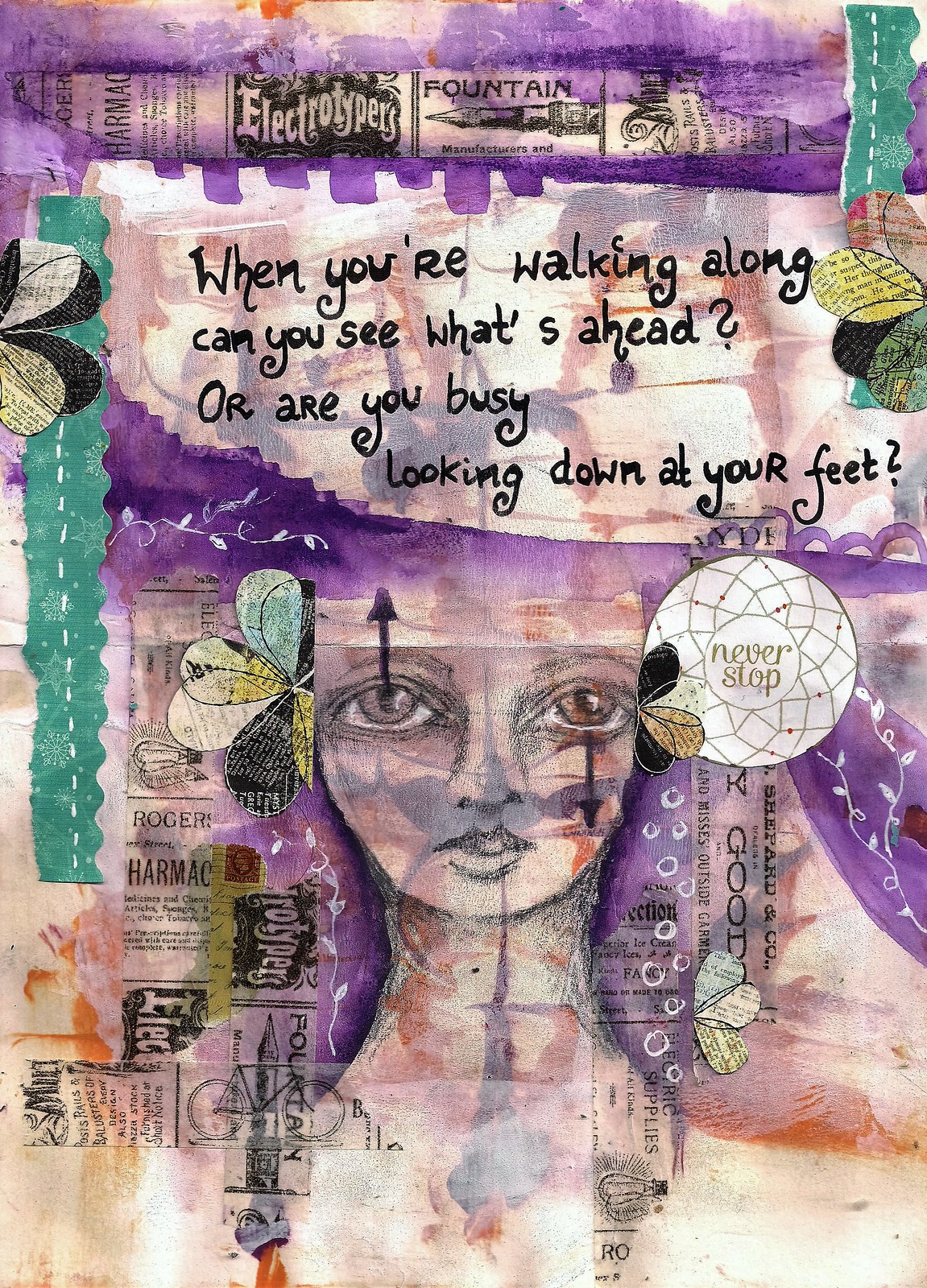The image is a vibrant and multi-colored artistic collage, brimming with various elements and details. Dominating the center is a drawing of a young woman, depicted from her neck up, showcasing pronounced facial features with large eyes, a distinct nose, and mouth. Surrounding her head are what appears to be flower petals, as if they are adorning her hair. To the side of her face, there is an oval white shape inscribed with the motivational phrase, "Never Stop."

At the top of the collage, a series of book spines are partially visible, featuring titles like "Electrotype" and "Fountain," though not all are legible. A prominent piece of black text in handwritten style asks, "When you're walking along, can you see what's ahead? Or are you busy looking down at your feet?" This question adds a thought-provoking, reflective tone to the piece.

The rest of the poster is an eclectic mix of colors and elements: swaths of purple, green, and off-gold, along with spots, petals, and fragments of newspapers and magazines. Notably, in the far upper left corner, a couple of dragonfly wings can be spotted, adding to the whimsical nature of the artwork. A blue, black, and yellow butterfly also adds to the collage's richness. The entire composition exudes creativity and inspiration, encouraging viewers to ponder and look forward.